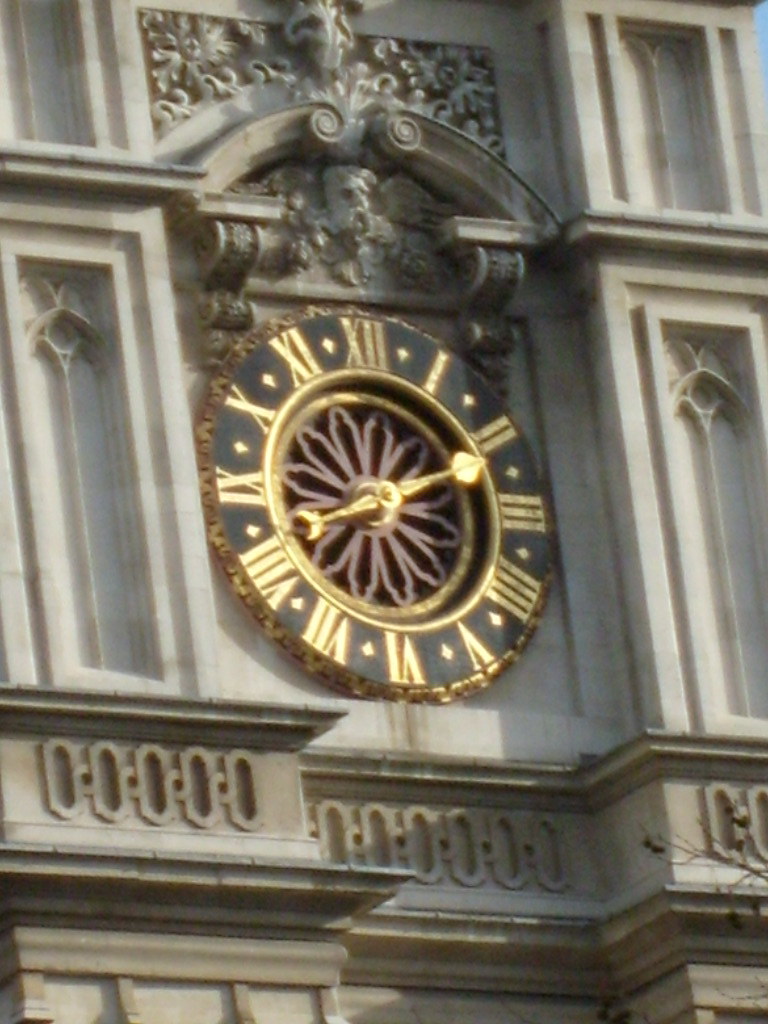The photograph captures a prominent, ornate analog clock affixed to the side of a historic stone building, possibly a church or government structure, known for its old architecture. The clock face is proportionately tall, about 20% taller than its width, with an encompassing black background. Its timekeeping features include gold hands and Roman numerals, also in gold, precisely positioned around the periphery. Between the numerals, there are diamond-like markers, adding a touch of elegance. A unique, repeated purple silhouette resembling a men's room symbol encircles the clock hands, giving an impression of flower petals radiating outward. The middle section of the clock displays a subtle bronze hue. The backdrop of the clock is a decorative stone wall adorned with archway carvings and spiral patterns, accented with small circular motifs towards the lower middle part. The close-up perspective emphasizes the clock, leaving much of the building's intricate stone patterns and textures only partially visible, yet showcasing the building's grandeur and fine craftsmanship.